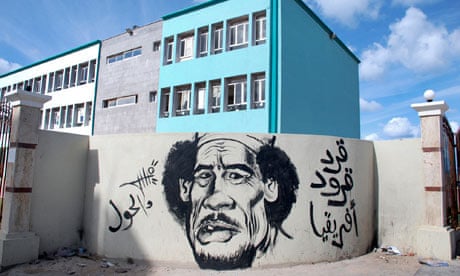The photograph captures an outdoor scene in broad daylight, possibly in Kuwait, showcasing a large building with distinct sections painted white, gray, and light blue. In front of the building stands a curved wall that features a vivid piece of graffiti art depicting an older man with black hair, possibly Saddam Hussein, with a cigarette in his mouth. Accompanying the portrait is text written in a non-English language. The sky above is dotted with white clouds against a backdrop of blue. To the left, the wall concludes at a gate, while to the right, it ends with a pillar topped by a ball. The urban environment appears somewhat barren, further highlighting the striking graffiti and the colorful building behind it.